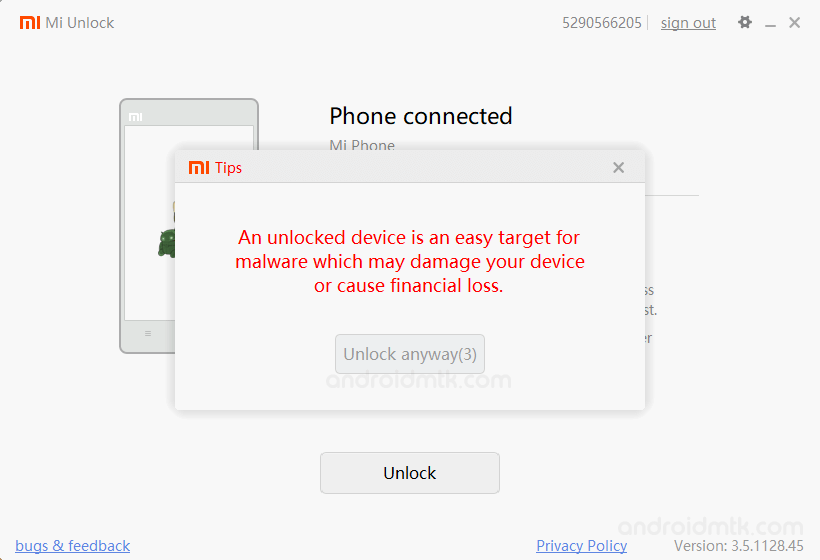The image shows a light gray background with various elements and texts arranged across it. In the upper left-hand corner, there is a slightly darker gray text that reads "MI" followed by "Unlock." To the right, there is a sequence of numbers "5290566205" and an underlined "Sign Out." Next to this text, there is a gear icon along with a gray underscore and an X.

Overlaid on the background is a rectangular pop-up window. The top border of the pop-up is gray. In the upper left corner of the pop-up, the word "Tips" appears in red text, while the upper right corner has a gray X for closing the window. The main body of the pop-up has a white background with a red warning message that states, "An unlocked device is an easy target for malware which may damage your device or cause financial loss." Below the message is a gray rectangle, and inside it, in darker gray text, reads "Unlock Anyway" with "(3)" in parentheses.

Outside of the pop-up, there is another gray, rectangular box that contains the word "Unlock" in black text. At the bottom right corner of the image, "Privacy Policy" is displayed in blue text, and on the left side, also in blue text, "Bugs & Feedback," both of which are underlined. In the lower right-hand corner, gray text reads "Version 3.5.1128.45," placed above "Android MTK," hinting at a likely website reference ending in ".com."